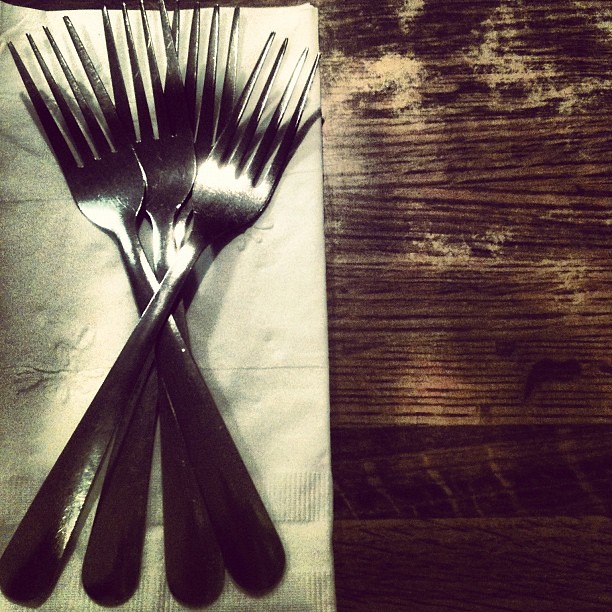This detailed close-up photograph captures four shiny silver forks arranged in a crisscross pattern, resembling a layered "X" formation, with their tines fanned out and handles overlapping. The forks are laid out on a white napkin that features subtle flower embossments and ridges at the bottom. The napkin, neatly folded, is placed on a dark, worn wooden table, showing visible grains and marks from usage. The lighting in the image is dramatic, enhancing the shadows and creating a high-contrast effect that makes the blacks appear more pronounced while the overall image is slightly darker. The right half of the photo showcases the textured wooden surface, while the left focuses on the napkin and forks, creating a visually balanced composition.